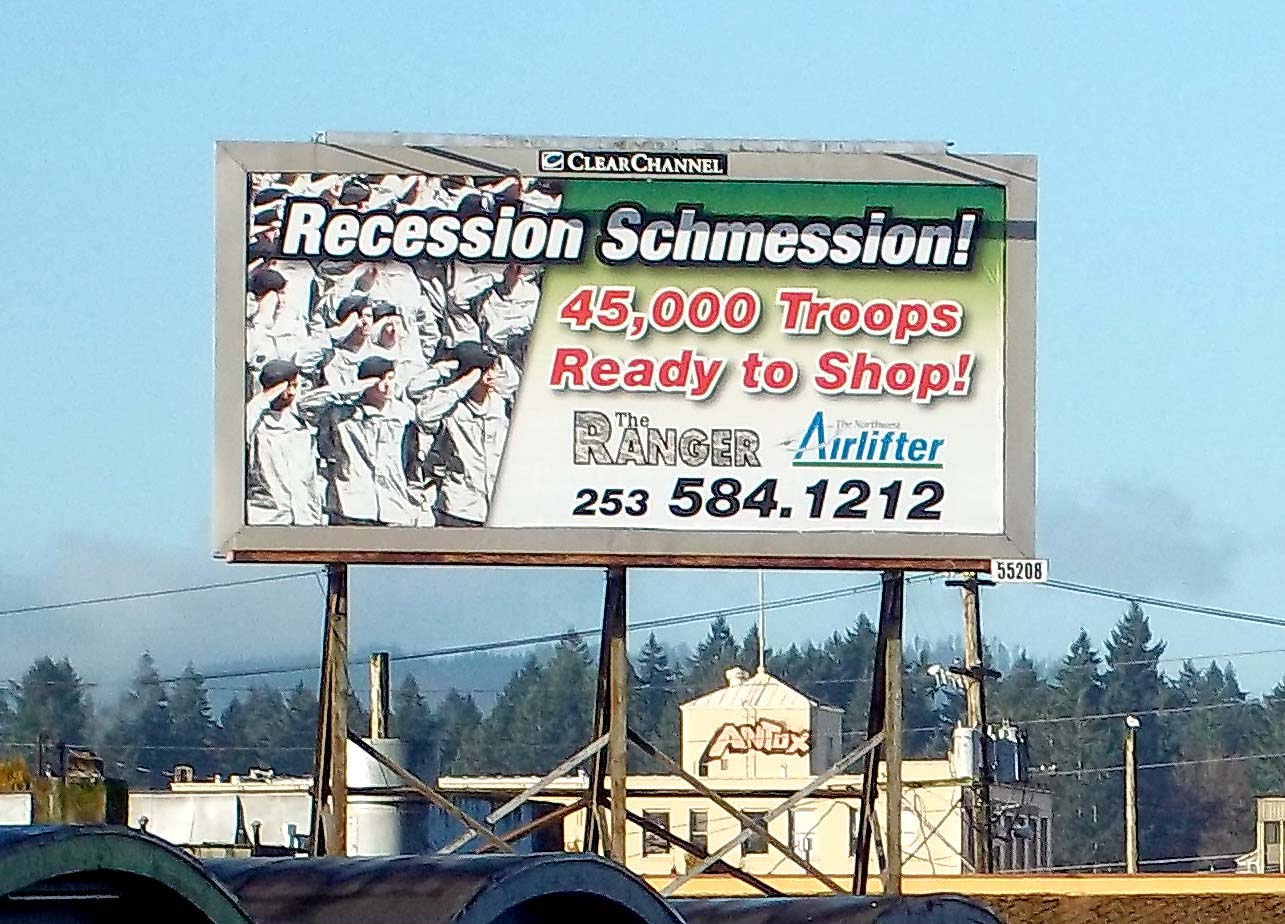This color photograph features a prominent billboard situated against a clear, blue sky with occasional small gray clouds near the bottom. The billboard itself is encased in a gray frame, giving it a picture-frame style. At the top center of this frame is a logo consisting of a small rectangle with a 'C' inside, pointing to the top right, next to the words "CLEAR CHANNEL" in all capital white letters on a black background. The focal content of the billboard includes a left-side image of numerous soldiers saluting, clad in gray uniforms with black hats. Above them, bold white text reads, "RECESSION SCHMESSESION!" Below this, in striking red lettering, it states, "45,000 TROOPS READY TO SHOP!" Towards the lower right section, on a green background that transitions into white, are the names "THE RANGER" in gray and "THE NORTHWEST AIRLIFTER" in blue, followed by the phone number "253-584-1212."

In the backdrop, there's an industrial-style building or possibly an old factory or school, topped with a smaller structure and a large antenna. The building's second story bears spray-painted graffiti reading "ANTOX" repeated twice. Numerous power lines stretch across the scene, supported by a power pole to the building's right. In the distance, a dense line of fir trees is visible, suggesting the photo was taken during daytime.